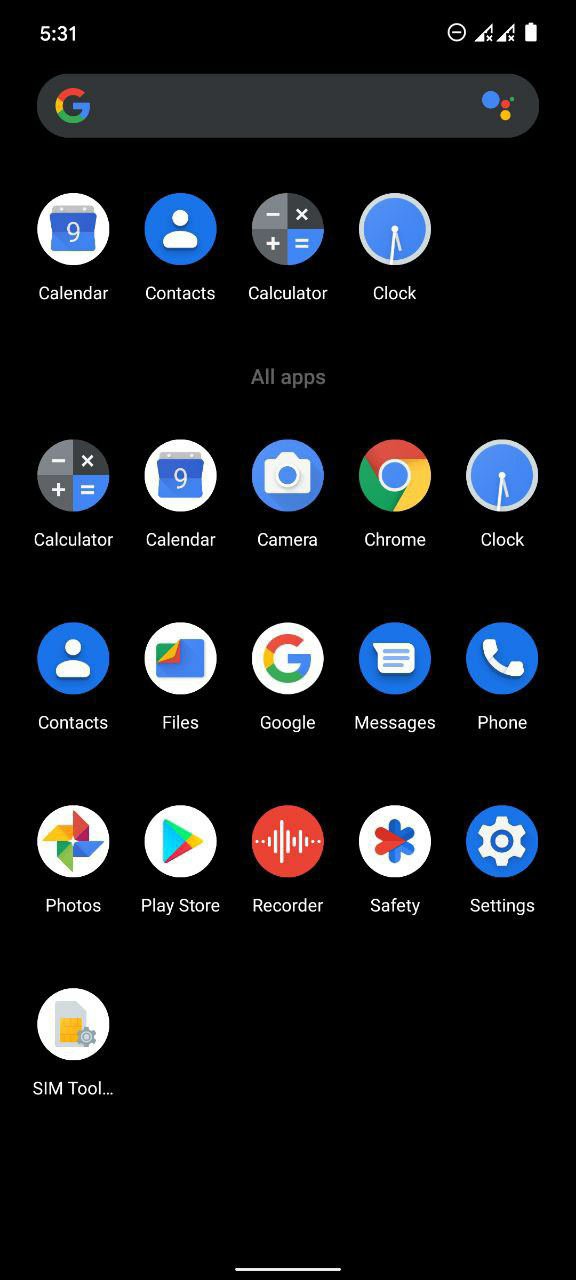This image is a screenshot of an Android mobile device's home screen. In the top left corner, the time is displayed as 5:31. To the top right, several icons are visible: the Do Not Disturb icon, network signal indicators for SIM 1 and SIM 2, and the battery level indicator. The screen features a collection of app icons neatly arranged, including Calendar, Contacts, Calculator, Clock, Camera, Chrome, Files, Google, Messages, Safety, Settings, Recorder, Play Store, SIM 2, Photos, and Files. This snapshot effectively showcases the device's current interface and available applications.